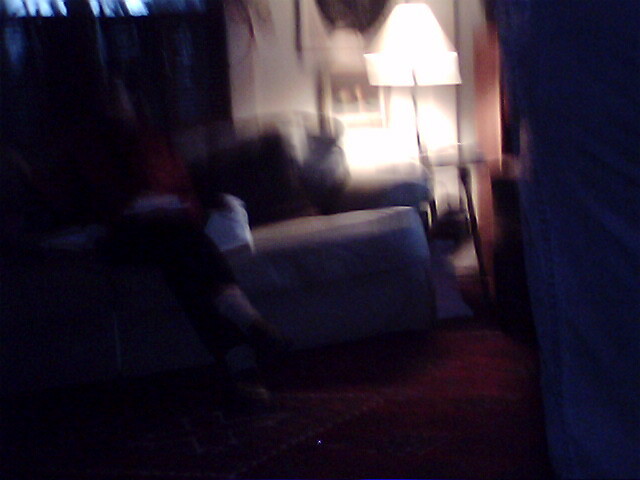A blurred and out-of-focus image captures a cozy living room setting. In the foreground on the right, a portion of a person's leg clad in blue jeans is visible. The carpeted floor has a red base with a large white diamond pattern in the center, containing a smaller white diamond within it. The background features a gray couch with two crossed legs clad in dark pants, suggesting someone is seated, though details are unclear. On the arm of the couch, there seems to be a cat perched comfortably. A distinctive lamp with a conical shade—smaller at the top and wider at the bottom—is positioned off to the side. The background wall is white, complemented by dark blue or black curtains hanging in the back left corner of the room.